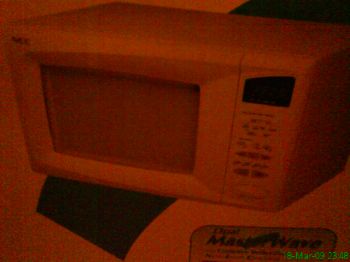In this dimly lit, predominantly dark orange and black image, we see a white rectangular microwave oven that appears to be part of an advertisement. The microwave, positioned atop what seems to be a countertop, is reminiscent of older, compact models with a capacity of around 0.5 or 0.7 cubic feet. The control panel, located on the right side, features numerous pressure point buttons and a slightly slanted, dark display screen, indicating it is an older design. Additionally, there is an unidentifiable brand name in the top left corner. Beneath the microwave in the advertisement is a black square, possibly a shadow or a black towel. A timestamp in neon green at the bottom right corner records the date as the 8th of March 2009 and reads "23 AP," indicating when the photograph was taken. The overall scene feels enclosed under a reddish-orange tent-like lighting.